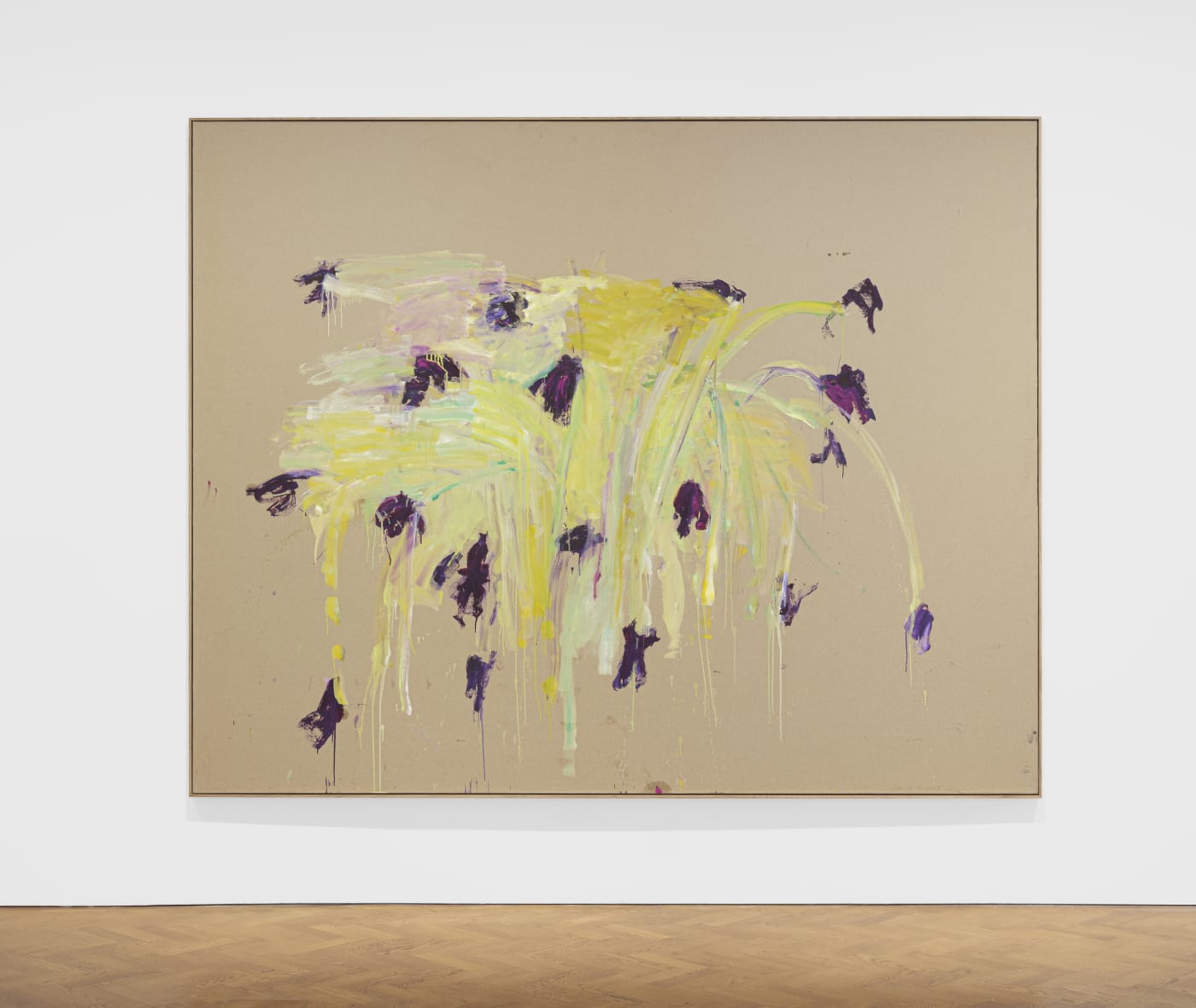The image depicts a photograph of a painting hung on a white wall, possibly in an art gallery. The painting is on a brown canvas with a very thin, barely noticeable black or dark frame. The floor beneath the painting is brown and featureless. The painting itself is highly abstract, featuring a tan background. Dominating the composition are vibrant strokes of yellow paint, interspersed with small purple blobs. The yellow paint sprawls out in various directions, giving an impression of movement or splaying. At the tips of these yellow strokes, the purple blobs appear, possibly resembling flowers or petals, hinting at a natural theme. This abstract painting may evoke images of a plant or flowers, with some interpretations suggesting a scene of wilting or drooping blooms, while another perspective sees the structure as a person dancing.